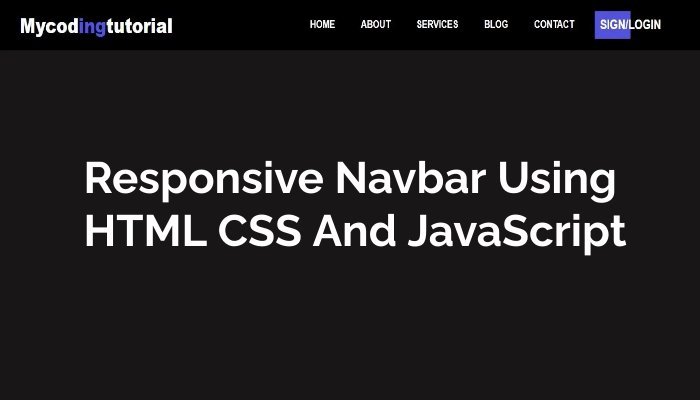The image is a screenshot from a computer display, depicting a coding tutorial website. The focal point is a horizontally-oriented black rectangle situated in the center, with white text in the middle that reads "Responsive Nav Bar using HTML, CSS, and JavaScript." In the upper left corner of the black section, it says "My Coding Tutorial," with the letters "ING" in "Coding" highlighted in purple, contrasting with the rest of the white text.

On the right side of the black rectangle, there's a horizontal navigation menu featuring clickable white text options that include: "Home," "About," "Services," "Blog," "Contact," "Sign In," and "Log In." The "Sign In" option appears to be selected, indicated by a purple rectangle outlining the word. The overall appearance is of a clean, well-organized web interface designed for users to follow along with coding tutorials. The image predominantly features a sleek, modern design with a black background and sharp white text, punctuated by subtle purple highlights for emphasis.